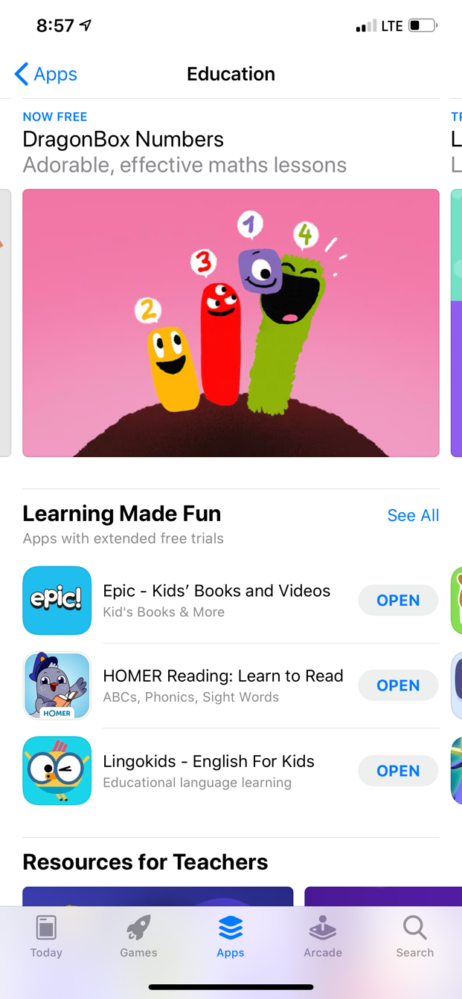**Detailed Caption:**

This is a screenshot of a Mexican educational app interface. At the top of the screen, the word "Education" is prominently displayed. To the left of this title, there is a "Back" arrow icon next to the word "Apps," both highlighted in blue. Just below, a blue-highlighted text reads "Now free." 

Further down, in bold black text, the app showcases "DragonBox Numbers." Underneath this title, a description in gray text states, "Adorable, effective math lessons." Below the description, an image depicts three numbered worms — green, red, and yellow — each with cartoon faces. These worms appear alongside a purple square creature, also with a cartoon face, peeking out from what seems to be a coconut shell or the ground, all set against a pink background.

The caption under the image reads "Learning made fun, apps with extended free trials," with the word "All" appearing in blue text on the right. Beneath this section, three other educational apps are listed: "Epic Kids Books and Videos," "Homer Reading: Learn to Read," and "Lingokids English for Kids." Each app listing includes a gray "Open" button with blue text, positioned on the right side.